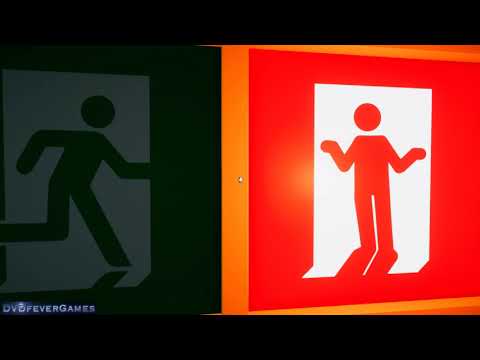The image is a detailed computer graphic with a predominantly black background, featuring two pedestrian-style figures reminiscent of street or instructional signs. Across the bottom and the top of the image, there are black bands. In the bottom left corner, very small blue lettering reads "DVD Fever Games." 

On the left side of the image, the first graphic shows a stick figure, similar to one seen on a street sign, running towards the right. This figure, depicted in a simplistic, black, and gray design, has a circular head floating above a neckless body, with one arm outstretched and the other trailing behind. The figure is enclosed within a black border rectangle.

To the right, the second graphic features another simplified stick figure set against a light orange border with a darker orange background. This figure stands within a white rectangular "doorway" and has an orange hue. The figure faces straight ahead, holding both hands up at shoulder level in a shrug, conveying a sense of confusion. The ground beneath it shows the figure's legs casting a shadow onto the floor within the doorway. Repeat details emphasize the contrasting design elements and the distinct poses of the two figures.